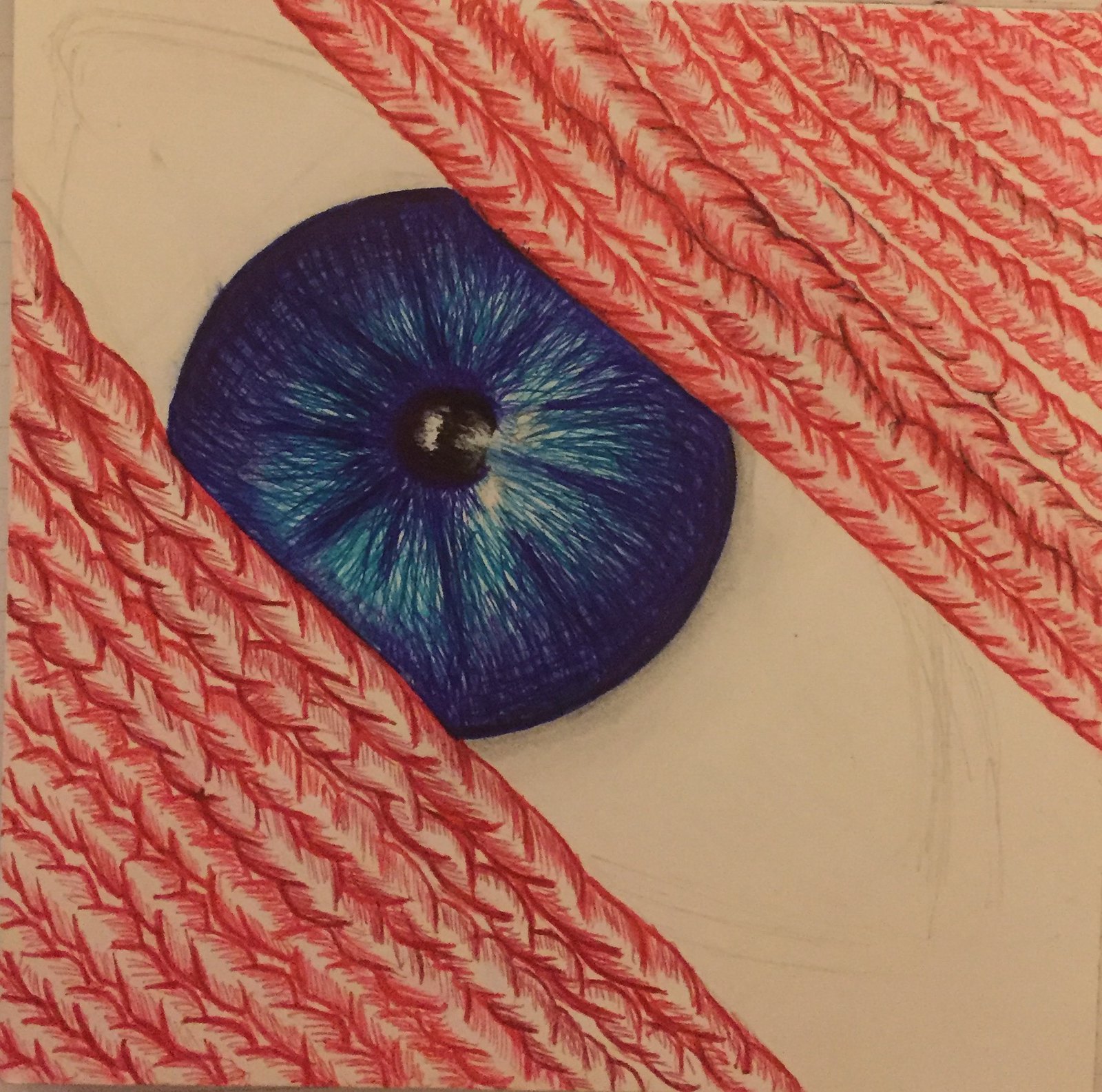The image is a detailed, computer-generated drawing designed to resemble a sketch. It is a square artwork dominated by a sandy beige background. Diagonally crossing the image from the upper left to the lower right is a central beige swath. This swath bisects diagonal, ropey-looking red cross-hatchings at the top right and bottom left corners, forming triangular patterns. These red elements resemble braided fabric, giving the appearance of a textured material, possibly a pillow or blanket. At the center of the image, partially obscured by the red ropey patterns, is a circular blue object that resembles an eye or a round pillow with a gathered center. The "eye" has a dark perimeter, brightens toward the middle, and features a small black dot at its core. The red cross-hatching overlaps the blue circular object, concealing parts of its edges, creating a layered and intricate composition.